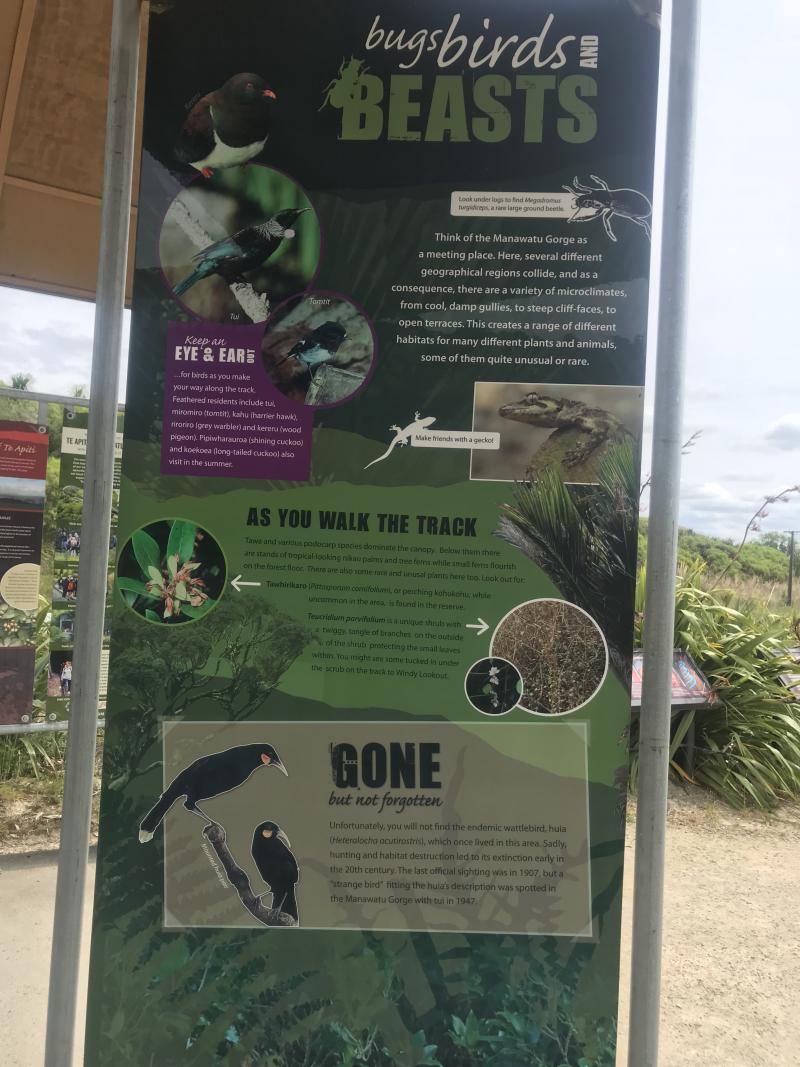The image depicts a zoomed-in view of an informational sign outside. The sign, held between two metal posts only partially visible within the frame, resembles something you might find at a zoo or a nature trail. The central theme of the sign is "Bugs, Birds, and Beasts," displayed prominently in white text against a dark green to almost black background. Below this title, there are various sections with photographs and text descriptions of different wildlife.

At the top left of the sign, three bird images are featured. One is a dark bird with a white breast and an orange bill. Another bird is highlighted within a circle, as is a smaller bird in a similar spotlighted circle. Accompanying text in this section urges visitors to "keep an eye and ear" on these birds, though some words are unreadable.

Moving down the poster, visitors are informed about different species they can expect to see. There is an image of a bug, potentially a cockroach, with accompanying information on the creature. A little lizard and a snake follow in the visual lineup, each with their own descriptors.

Text further down the sign reads, "as you walk the track," suggesting an educational journey through the area. At the very bottom, a poignant message states, "gone, but not forgotten," below which are images of two black birds with a distinct pink spot under their eyes, symbolizing extinct animals. 

The background surrounding the sign consists of green trees, leaves, and bushes, suggesting a natural, outdoor setting. To the left, more signs and vertical poles are faintly visible, along with the edge of a wooden roof structure. The ground, primarily dirt, complements the rustic, educational ambiance of the scene.